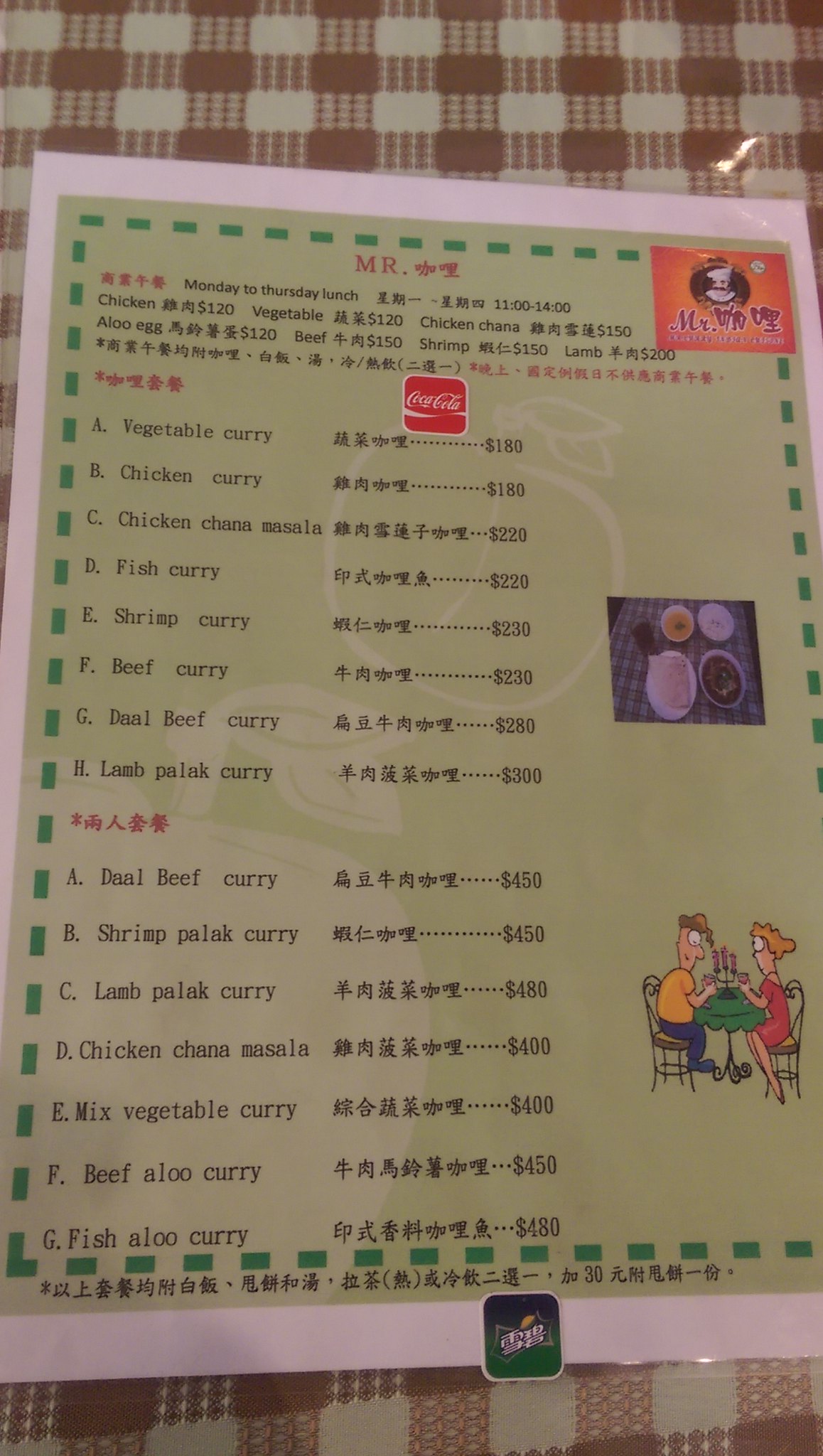This photograph captures a detailed view of a menu set against a slightly reflective surface characterized by a white and reddish-brown design. The menu itself is bordered in white, followed by a decorative line of green dashes that outline a light grayish-green section.

At the top of the menu, just below a dashed green line, the words "Mr." appear in red letters alongside some Oriental characters. An orange square in the top right corner of the menu also features the word "Mr." in red letters, accompanied by the same Oriental characters, some indistinct letters, and a depiction of a man with a white chef's hat and a thick mustache.

Underneath the initial red lettering, written in black, the menu states "Monday to Thursday lunch" followed by Oriental characters and the time frame "11 o'clock - 14 o'clock." The menu reveals an assortment of dishes such as chicken, vegetable, chicken chana, aloo egg, beef, shrimp, and lamb, all accompanied by corresponding Oriental characters. A white and red square symbol featuring the classic Coca-Cola script is also present.

Further down, the menu lists additional items and includes two illustrations. One illustration is an overhead photograph showing three round bowls and a skillet filled with food. The other is a cartoon-style drawing of a man and a woman dining at a green table adorned with a three-pronged candelabra holding pink candles, while they sit on wrought iron chairs.

At the very bottom of the menu, there is a blue and green square symbol containing what appears to be an image of a lemon or lime along with some Oriental characters, likely representing the Sprite brand in a non-English script.